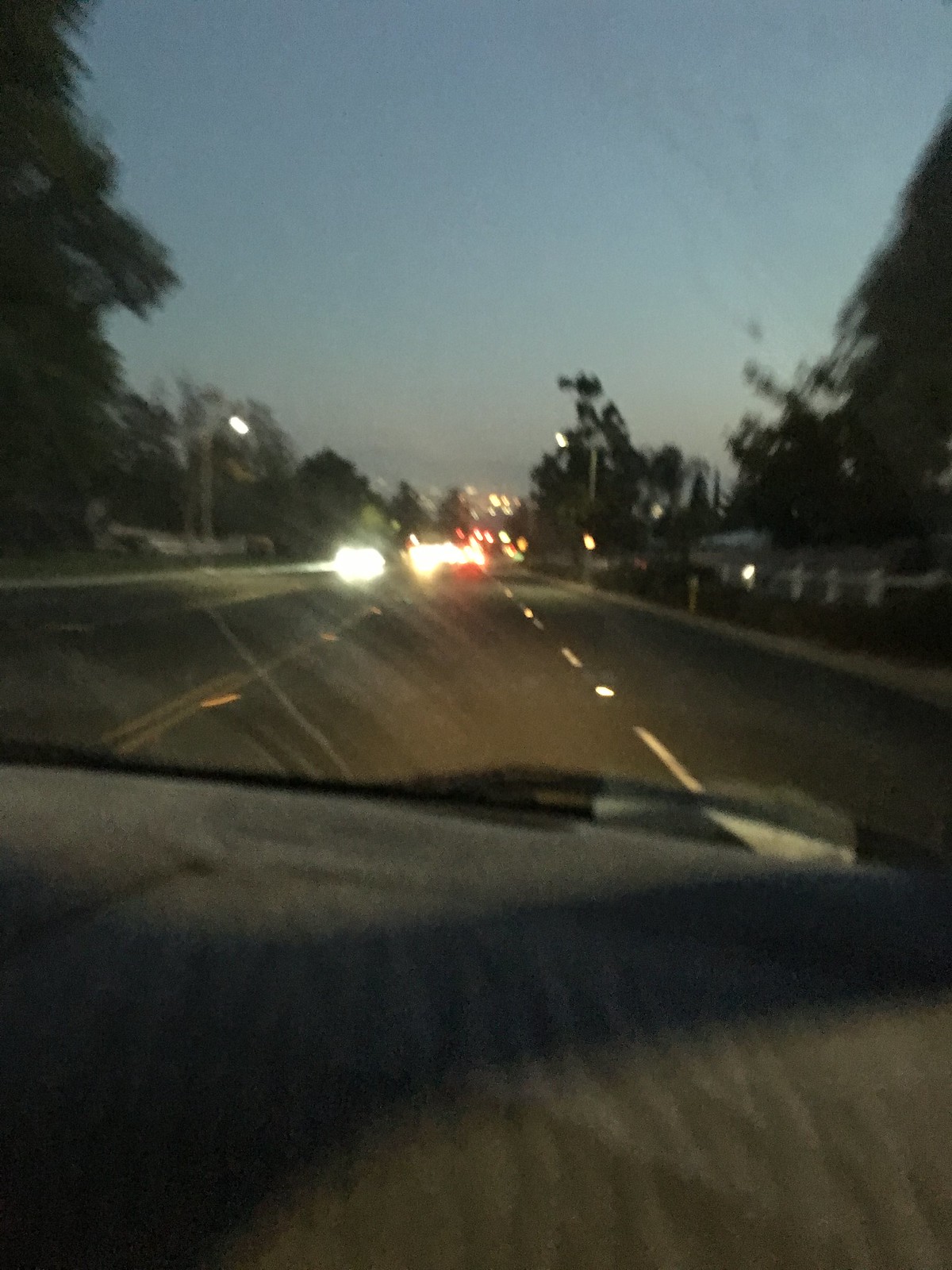A photograph captures the view from the passenger side of a moving car, looking through the front windshield. The gray dashboard is partially visible in the lower part of the frame, while a black windshield wiper rests outside on the glass. Light hits the windshield, revealing some streaked lines across it. Above, the sky is predominantly blue with slight overcast patches. Both sides of the road are lined with lush green trees. The dark gray paved road stretches ahead, with cars approaching in the left-hand lane and others traveling in the same direction in the lane ahead. The headlights of the oncoming cars emit a yellow glow, while the red brake lights illuminate the vehicles in front.